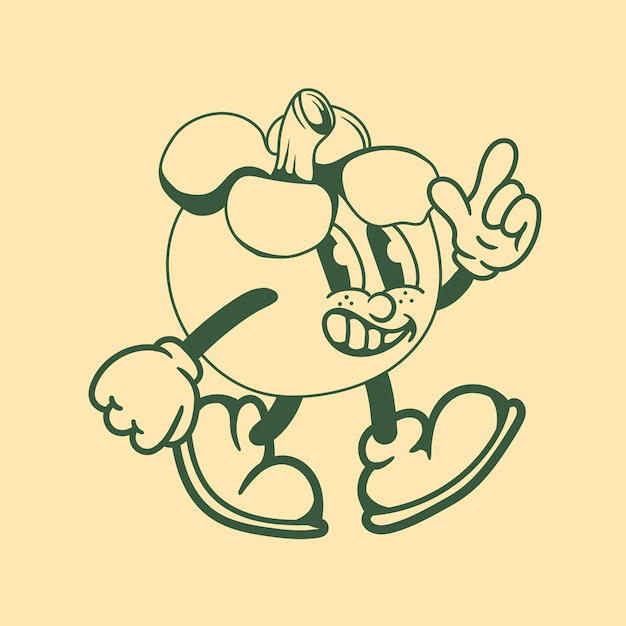The image depicts a charming, vintage-style cartoon character designed to look like an anthropomorphized fruit, most likely a tomato, given its rounded shape, freckled cheeks, and the stem and leaves at the top of its head. The character is illustrated using grayish-green lines, set against a peach-colored background. It has large, expressive comic book eyes, a nose, and a broad, happy grin. This fruit character features two arms, both wearing gloves; the right arm is hanging down by its side while the left arm is raised, with the thumb and forefinger forming a pointing gesture or finger gun. The character also has spindly black legs ending in big, chunky shoes, giving the impression that it is in mid-walk. The overall look, complete with vintage-style details like the gloves and big shoes, adds to the whimsical charm of this anthropomorphic fruit.